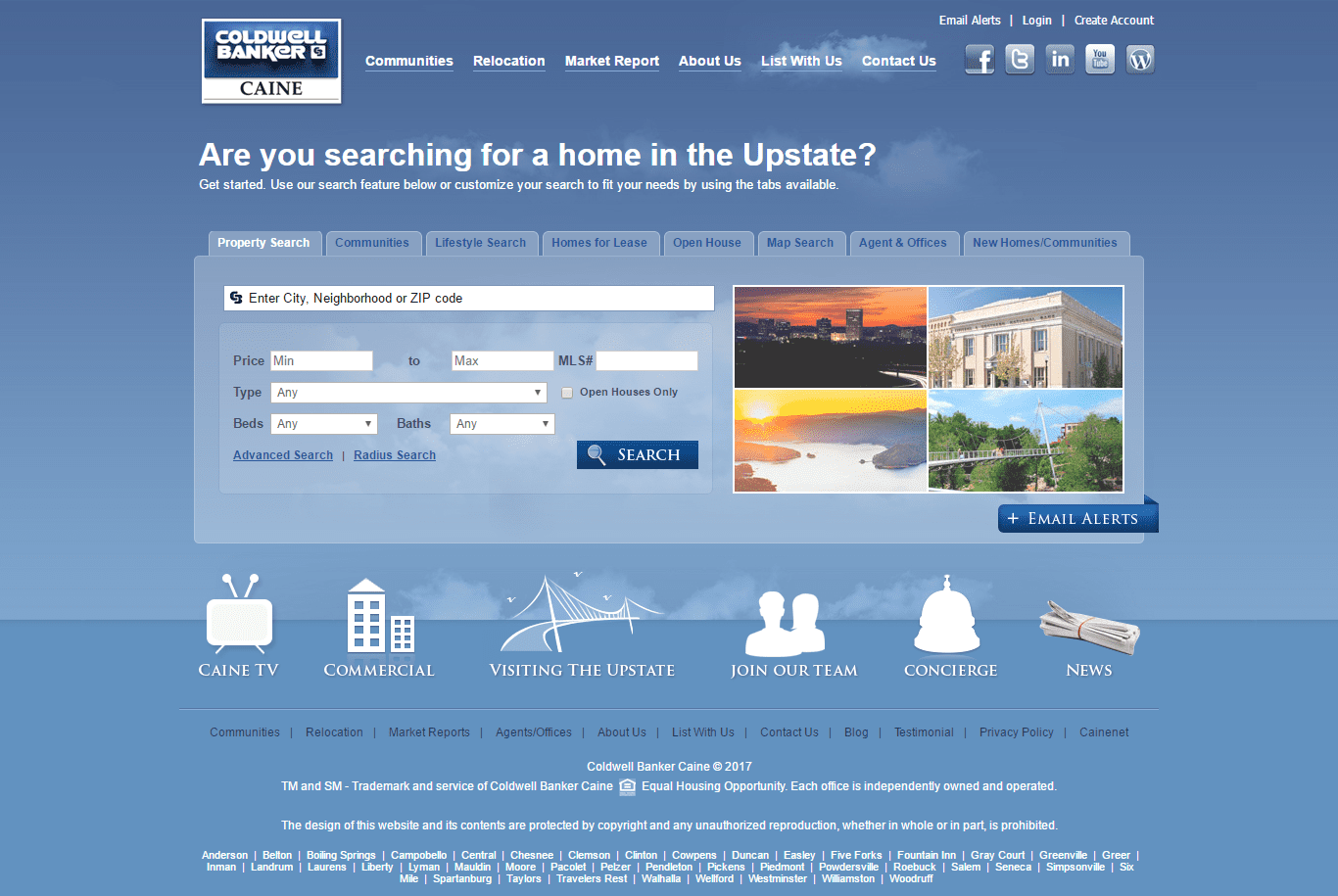Screenshot of Coldwell Banker's Online Portal

The image is a screenshot of the Coldwell Banker online portal. At the top left corner, the logo "Coldwell Banker" is prominently displayed against a blue rectangular background, with the word "Caine" (C-A-I-N-E) positioned just below it. To the right of the logo, a navigation bar features multiple tabs labeled as follows: Communities, Relocation, Market Report, About Us, List With Us, and Contact Us.

In the top right section of the page, there are additional options, including Email Alerts, Login, and Create Account. Right below these options, social media icons for Facebook, Twitter, LinkedIn, YouTube, and an unidentified platform with a "W" symbol are displayed.

Directly below the logo, a header poses a question: "Are you searching for a home in the upstate?" followed by a prompt to get started. It encourages users to utilize the search feature below or customize their search to fit specific needs by using available tabs.

The customizable search tabs include: Property Search, Communities, Lifestyle Search, Homes for Lease, Open House, Map Search, Agent and Offices, and New Homes and Communities. These options provide a comprehensive toolset for users to tailor their home search experience.